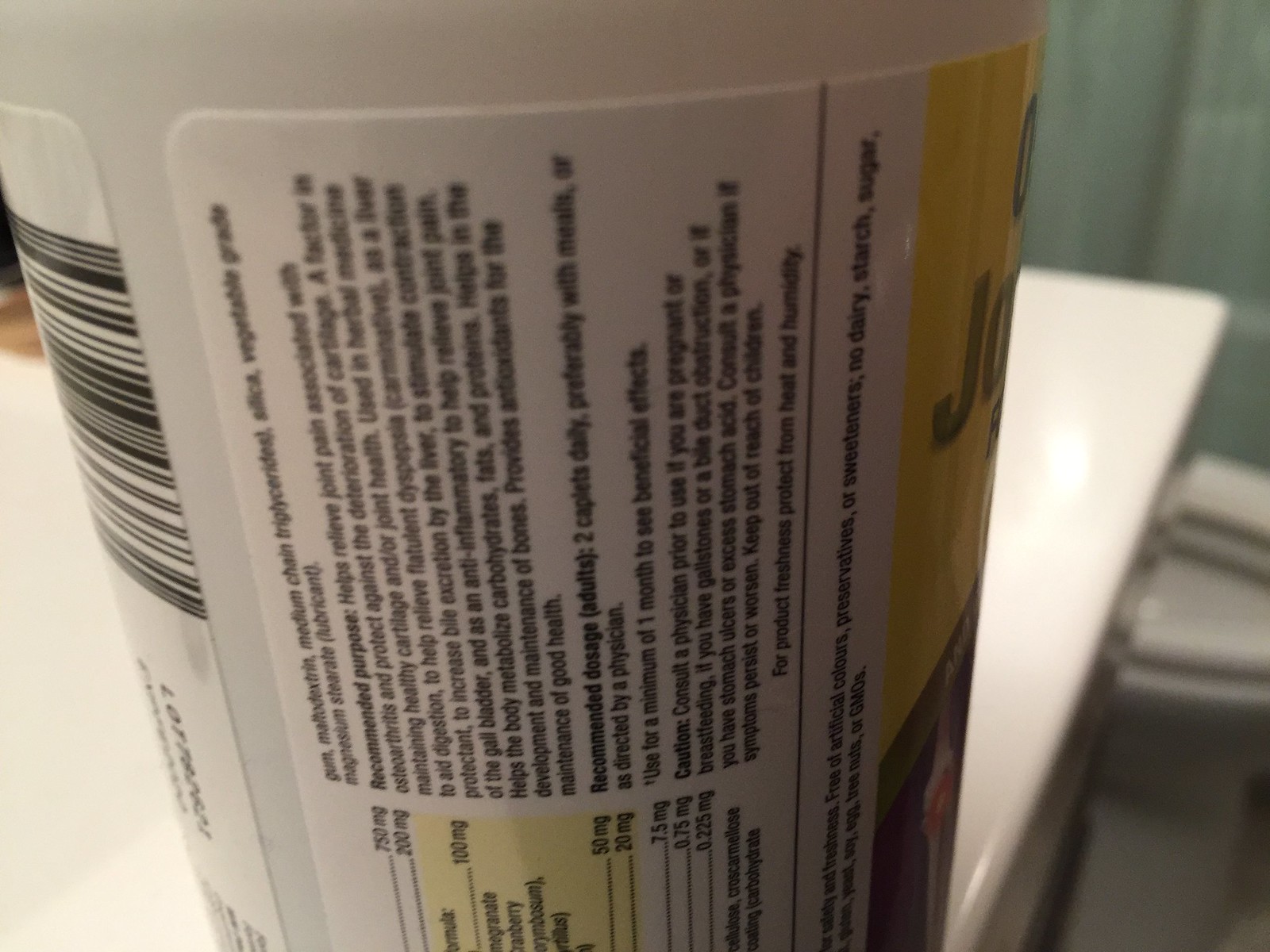A close-up photograph captures a label affixed to a bottle, detailing vital information about a dietary supplement designed for joint health. The label specifies a recommended dosage for adults: two caplets only, preferably taken with meals as per a physician's guidance. The product's primary purpose is highlighted as aiding in the relief of joint pain associated with osteoarthritis and providing protection against cartilage deterioration. Distinctively, a barcode is visible in the top left corner of the label. The label itself is adhered to the bottle without fully encircling it. On the right side, the label's yellow section stands out, listing the supplement's ingredients. The bottle is resting on a vanity counter, providing context to its placement and use.